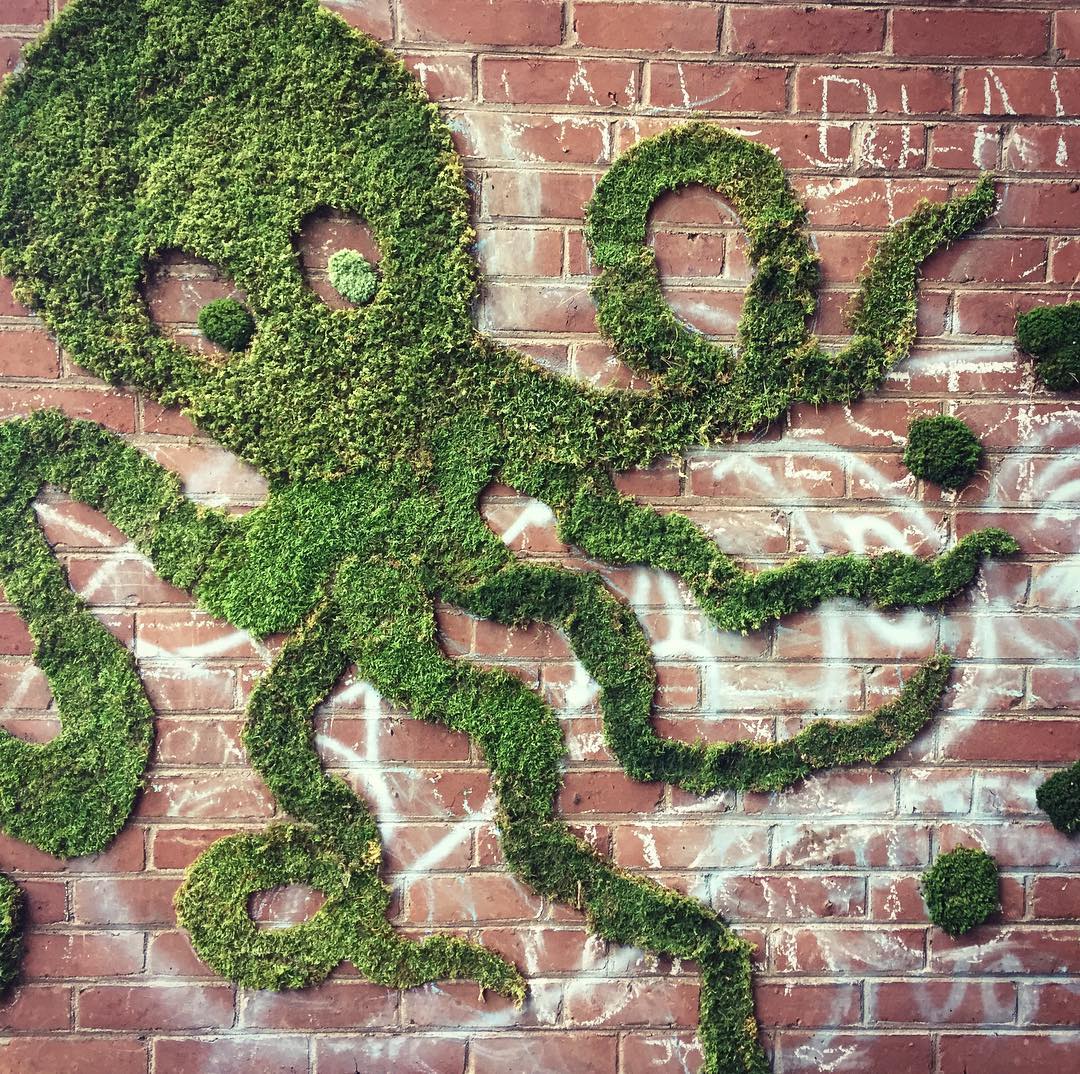This photograph showcases a brick wall of a light reddish, rusty color adorned with numerous indistinct white chalk drawings and letters, dusted and difficult to decipher. Dominating the scene is a striking green octopus crafted from moss, centrally positioned with its head angled to the upper left and its tentacles extending towards the lower left and right corners of the image. The octopus features two green eyes, fashioned from the moss itself, complete with pupils. Additionally, there are about four small moss dots to the right of the octopus, potentially representing bubbles. The overall visual effect is a vivid juxtaposition of the red brick and white graffiti background with the vibrant green moss art.